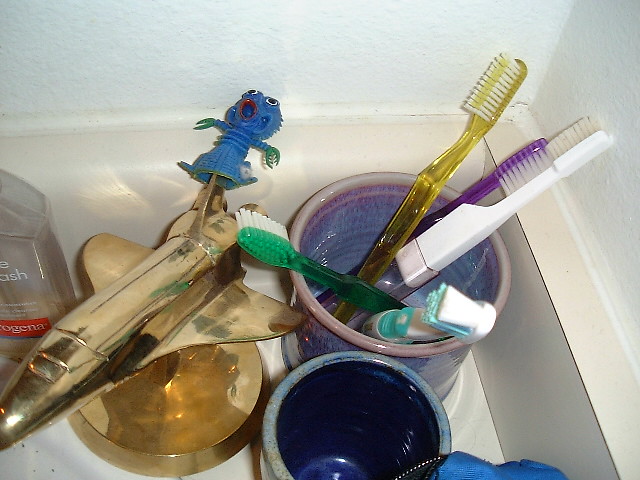This detailed photograph showcases a close-up view of a bathroom countertop corner, capturing a variety of personal and decorative items. The countertop, a beige color, meets a white wall at a 90-degree angle. Prominently featured is a purple ceramic cup holding five colorful toothbrushes with white bristles. These toothbrushes have handles in assorted colors: yellow, purple, white, green, and white-turquoise. Adjacent to the cup is an elegant gold paperweight shaped like a space shuttle, which sits on a circular base. Perched at the rear of the spacecraft is a vibrant blue toy creature with green hands, red lips, and wide-open white eyes, adding a whimsical touch. A bottle of Neutrogena face wash, nearly empty and mostly clear, stands to the left of the cup. In front of the purple cup and closer to the camera is an empty blue cup. Partially visible beside it is a piece of blue fabric. The overall composition, shot in landscape mode, provides a detailed and intimate glimpse into the everyday items arranged at the bathroom's sink area.